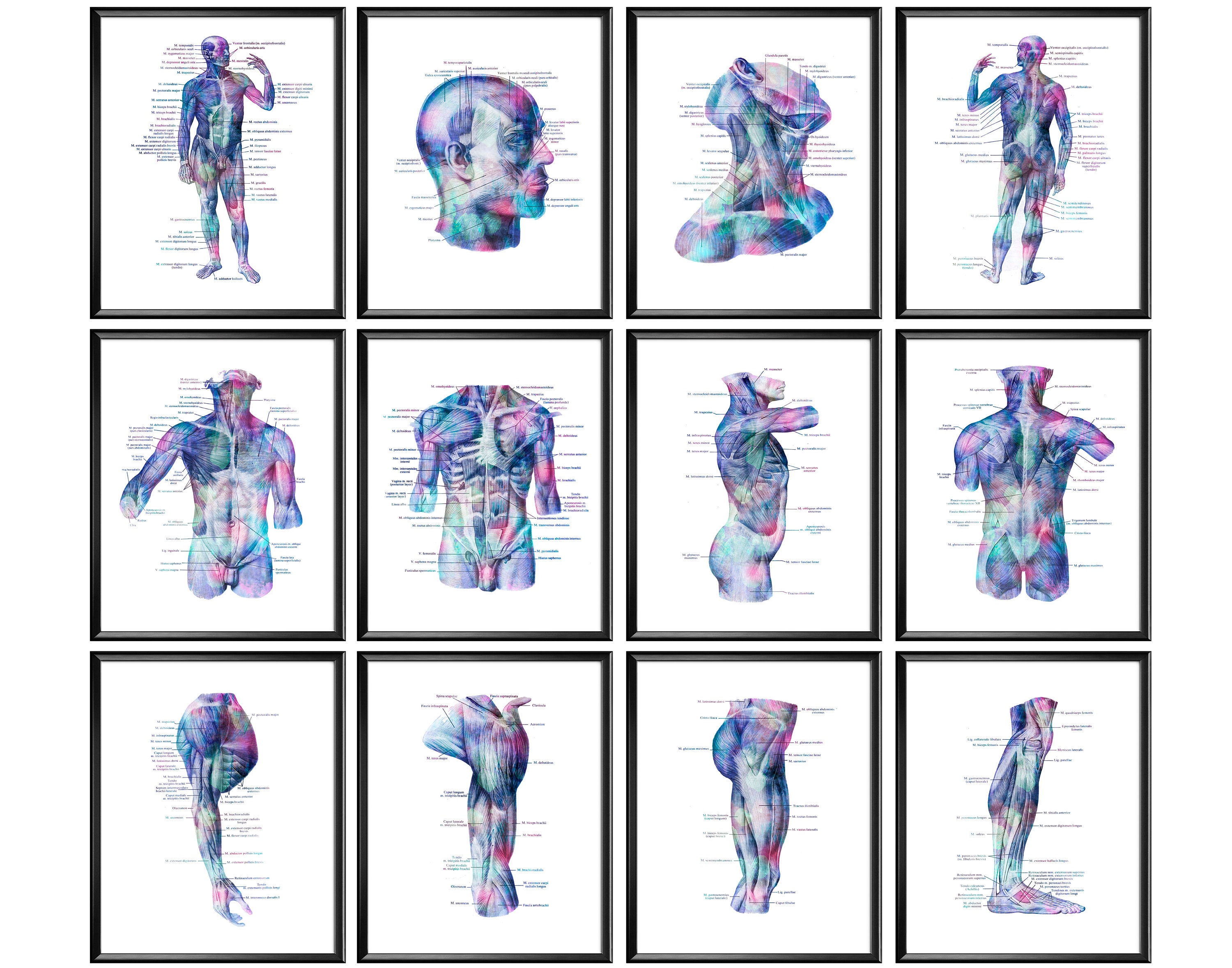The image depicts a collection of 12 framed, finely rendered human anatomy illustrations arranged in a 4x3 grid. Each illustration is outlined in black and separated by a small, half-centimeter gap. The stylized drawings are iridescent, displaying various shades of pink, turquoise, dark blue, white, and gray. Every piece features minute black labels indicating specific body parts, although the text is too tiny to read clearly.

The top row includes a full-body male figure standing with his right arm bent towards his mouth, a bald man's head facing slightly right, a drawing emphasizing the nasal cavity and ocular nerves with the head tilted back, and another full-body figure viewed from behind in the same pose as the first. The middle row starts with a close-up of the male torso down to the upper thighs with the left arm raised. This is followed by a similar torso view without the neck and forearms, a side view showcasing the extended right arm, and a rear view mimicking the previous side view but with the arm lowered. The bottom row features an upper torso with a relaxed right arm, a close-up of the forearm and shoulder, a segment of the thigh devoid of the foot, and finally, a detailed view of the lower leg from the knee down including the foot. All illustrations meticulously label various muscles and body parts, providing an intricate study of human anatomy.